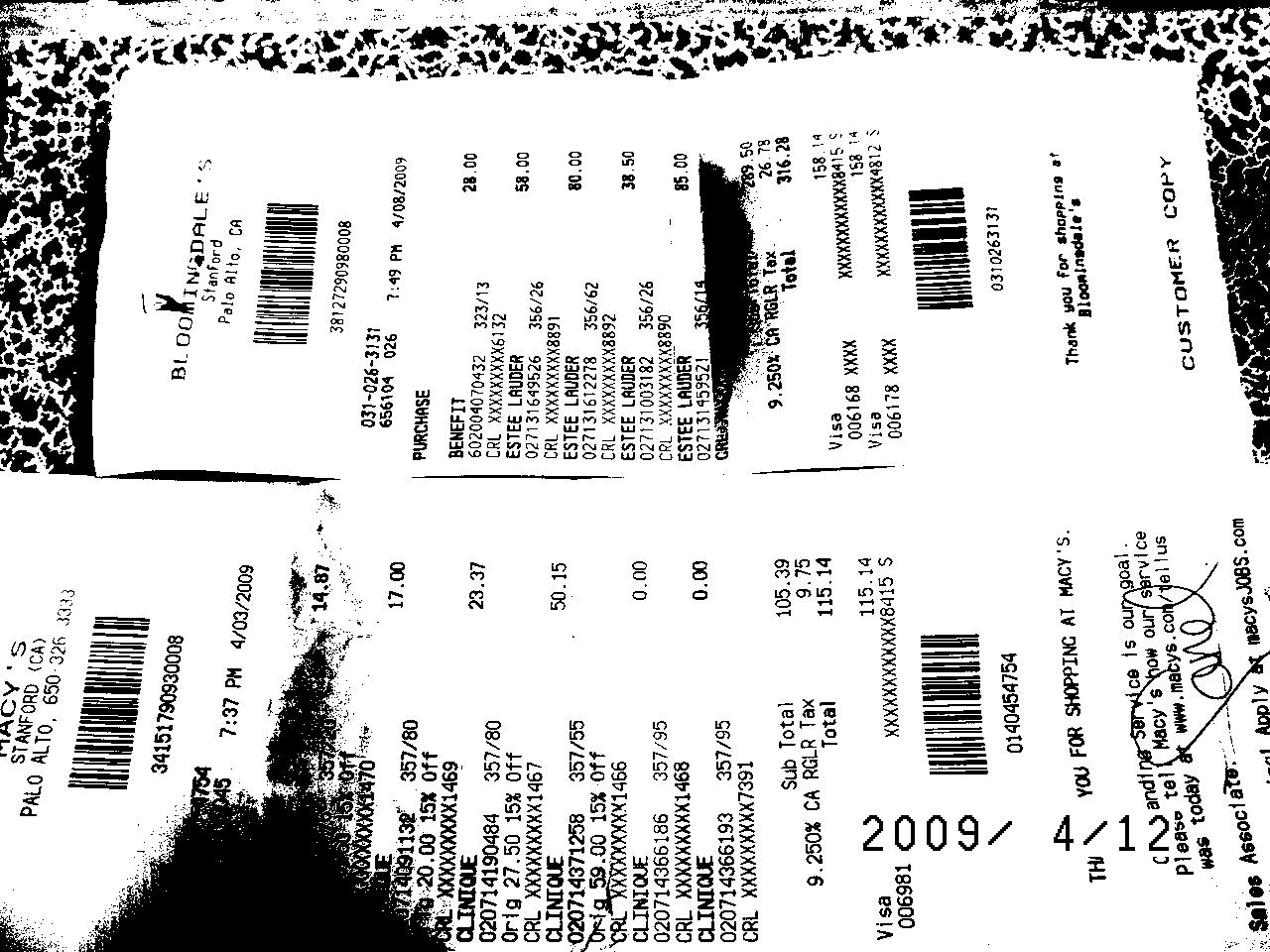The image displays two receipts from stores in Palo Alto, California. The first receipt is from Macy's, located in Stanford. Notable details include a contact number, which appears to be (650) 326-3333. The second receipt is from Bloomingdale's, also situated in Palo Alto. Both receipts indicate that the purchases were made using Visa cards, although it is unclear if the same card was used for both transactions. The receipts include itemized lists showing the purchase of products from brands such as Estee Lauder and Clinique. Both receipts also feature barcodes at the bottom and are marked "Customer Copy."